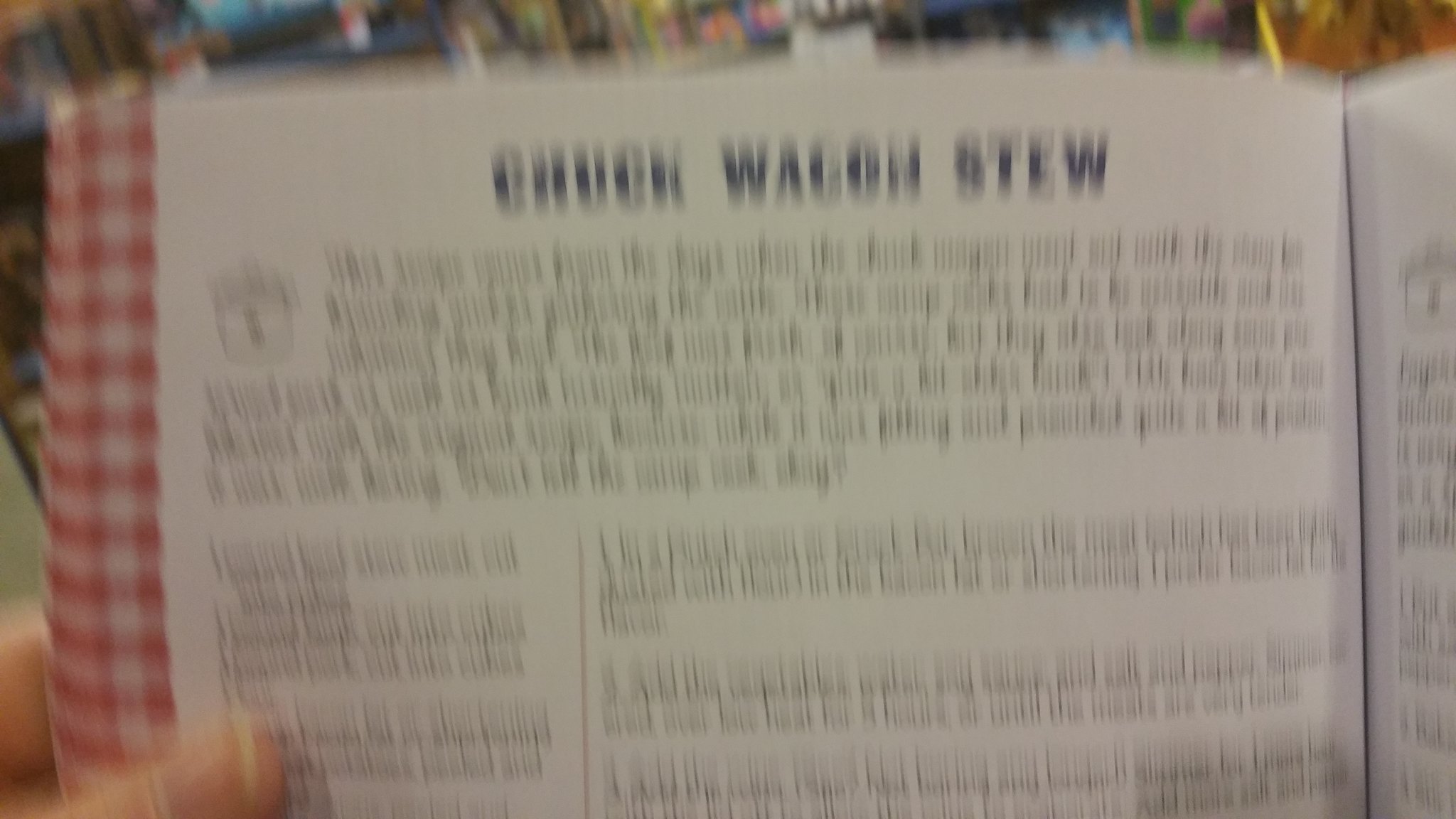The image is a blurry, digital photograph of a cookbook page held open by a person's thumb and forefinger. The background is a mixture of indistinct colors, including blues, greens, reds, whites, and a prominent orange on the right-hand side, suggesting it was taken indoors. The main focus is on the bottom left corner where the thumb is holding a page. The cover of the cookbook, featured on the left edge, displays a red and white checkered pattern with varying shades of red due to the overlap with the white. Despite the blurriness, the top of the page has big, bold black letters that read "Chuck Wagon Stew." Below this title, the text is illegible, but it appears to include a short description, possibly with a layout dividing ingredients on the left and recipe steps on the right. The page background is a cream color. The image overall suggests a hasty or accidental shot.